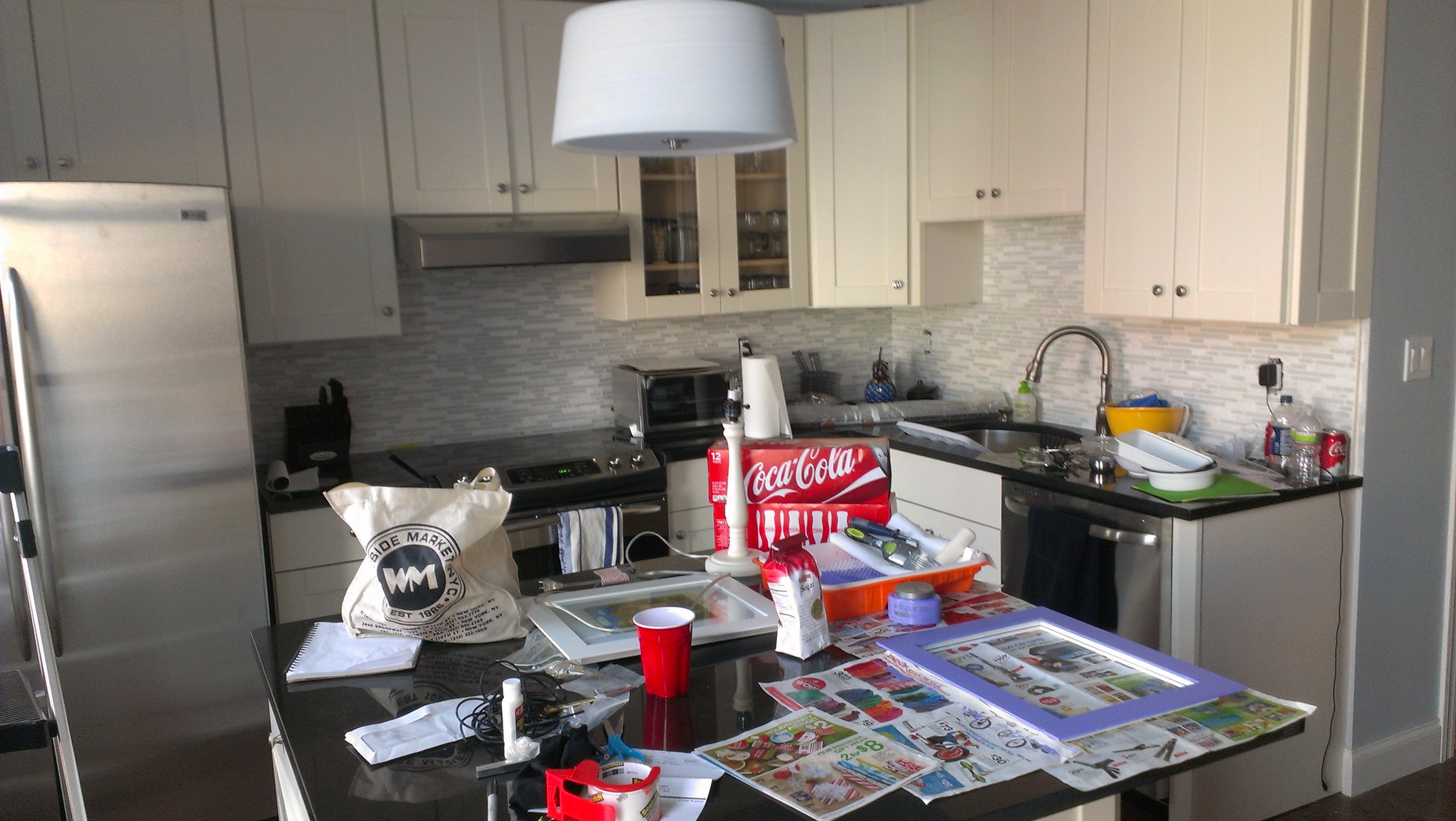This high-quality landscape-style photograph captures a modern kitchen featuring a central island adorned with black and colored granite countertops. Scattered across the island are several newspapers and a red Solo cup. On the island's top right corner, two twelve-pack boxes of Coke are stacked, and a khaki tote bag is positioned on the top left. To the image's left side, a stainless steel refrigerator is partially visible, cut off by the margin.

The kitchen showcases L-shaped light gray cabinets, with those in the corner featuring transparent glass doors. Below, there's an oven situated adjacent to the fridge, while a toaster is seen on the counter behind it. Further to the right, a dishwasher is positioned at the counter's far end. A cylindrical white lampshade, currently turned off, hangs above the scene. The backsplash is decorated with gray and white tiles, adding a stylish touch to the modern kitchen design.